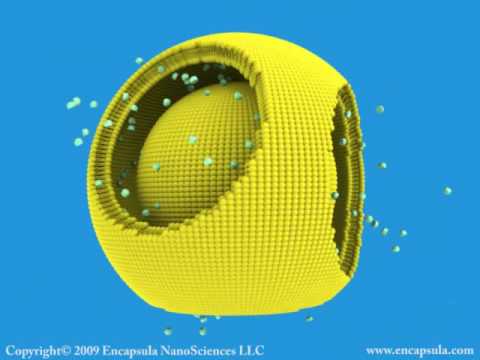The image depicts a digital graphic with a sci-fi feel, showcasing a spherical yellow structure set against a blue background, which evokes a sense of space or water. This yellow structure consists of two main components: an outer dome made up of tiny spheres that resemble foam, featuring two large round openings—one on the left and another slightly to the right. Inside this dome is a smaller yellow ball composed of similar tiny spheres. Scattered throughout the background are green and white particles, giving the impression of movement or energy. At the bottom left corner, the text reads "Copyright 2009 Encapsula Nanosciences LLC," and on the bottom right corner, the website "www.encapsula.com" is displayed.